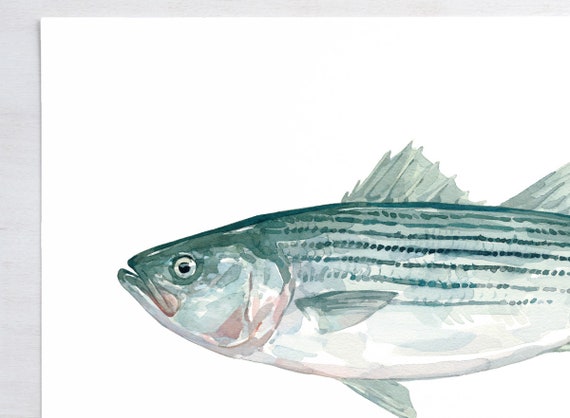The image features an artist's detailed rendition of a fish, showcased against a white background that appears slightly elevated at the upper left corner, mimicking a piece of paper mounted on the wall. The background has a gray border, with a thinner strip across the top and a thicker section along the left side. The fish is depicted in profile with its head facing the left and the tail end cut off, occupying at least half the paper’s width. It sports a green-hued body adorned with darker vertical stripes, a silvery-gray appearance, and a white underbelly. A touch of red near the head highlights the gill area, complemented by a black eye and a partially open mouth. The fish has several fins: a triangular, slightly jagged dorsal fin on top, a fin beneath its body, and a side fin. The scales are distinctly articulated, adding to the texture and realism of the drawing.